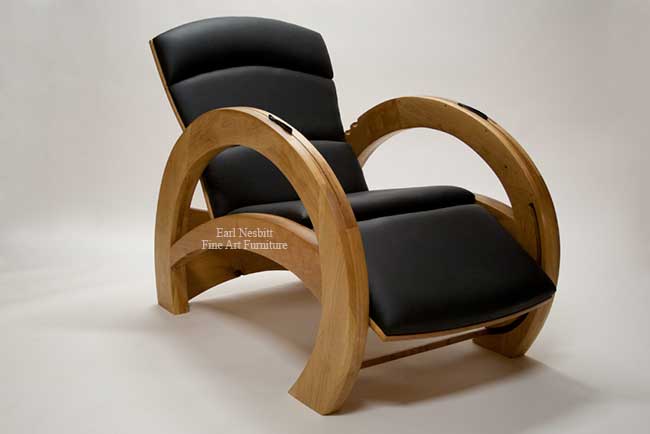This photograph showcases a distinctive lounge chair made of black leather upholstery with ridged padding. The chair features striking armrests that are uniquely C-shaped, crafted from a light, smooth wood that arches gracefully into a half-circle form, enhancing its elegant design. The wood is a light tan, further accentuating the sophisticated structure of the chair. The chair's frame includes a notable arch beneath the seat and a thin bar between the two front legs, with a wider piece of wood supporting the back. The overall shape of the chair is reminiscent of a stylized W, with a tall back that slopes down to a raised middle and recedes again towards the front, providing a comfortable reclined position. It is placed on a plain grayish-white background, creating a minimalist and clean aesthetic. The words "Earl Nesbitt Fine Art Furniture" are inscribed on the right wooden armrest, signifying its artisanal craftsmanship. This intricately designed chair combines both comfort and artistic appeal, making it an exquisite piece for any setting.